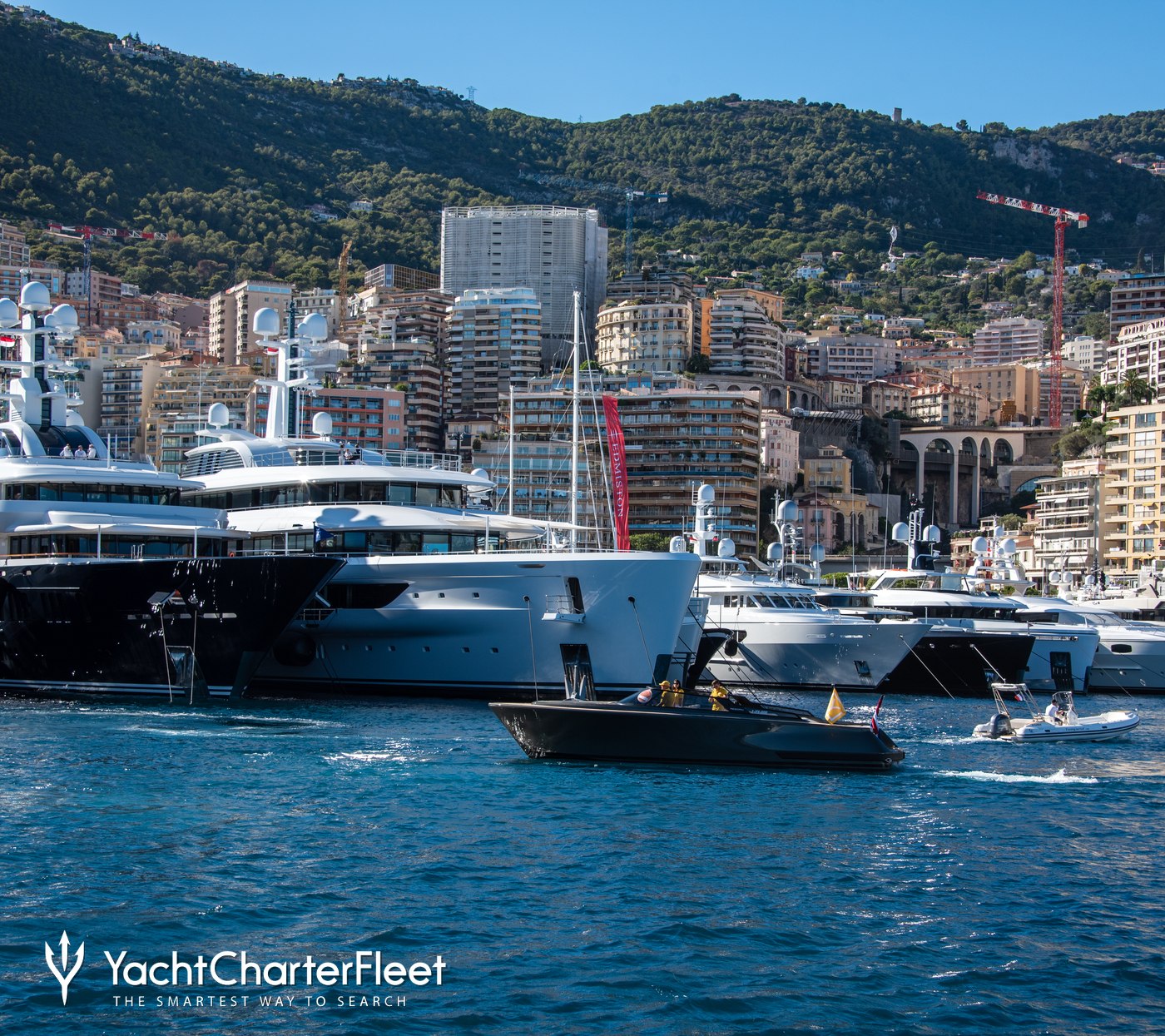The image vividly captures a bustling marina, likely in a Mediterranean or tropical coastal area, with the label "Yacht Charter Fleet" and the slogan "The smartest way to search" displayed prominently in white text at the bottom left, accompanied by a trident-like symbol. The scene is dominated by large, luxurious super yachts, including some white and a distinct black one, anchored alongside the dock. Smaller motorboats, including a noticeable small black boat with two people, float in the foreground against the blue waters. The marina is framed by a sprawling urban backdrop of densely-packed, multi-story buildings, possibly hotels or resorts, hinting at an affluent area. Beyond the cityscape, a verdant mountain dotted with trees rises, showcasing nature’s quiet contrast to the bustling waterfront. The clear blue sky overhead adds to the picturesque charm of this sophisticated harbor setting.